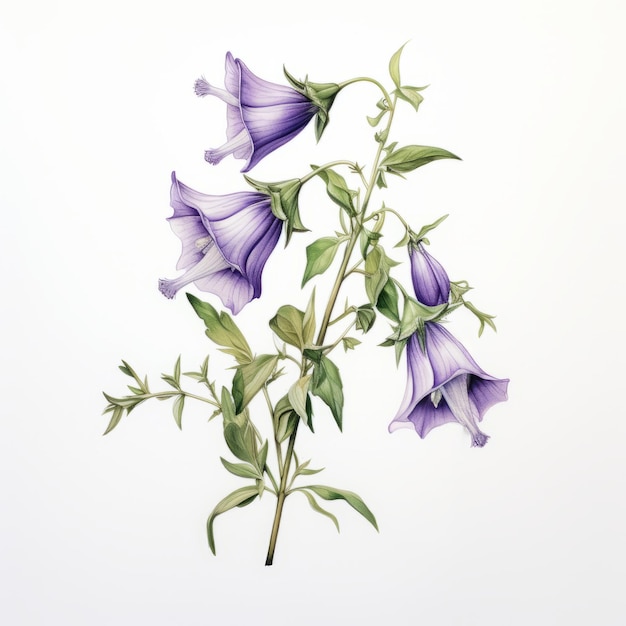This is a highly detailed illustration of a vibrant flowering plant, rendered with what appears to be colored pencils. The central stalk of the plant is a brownish-green color, from which multiple stems branch out, each adorned with lush, varying shades of green leaves. Four striking purple flowers in different stages of blooming are attached to these stems. The flowers, reminiscent of hibiscuses but uniquely shaped, boast intricate detailing with prominent stamens in their centers. Two flowers on the left are fully open, showcasing their bell-shaped petals accented with hues of purple and white. On the right, one flower is midway through blooming, while another remains a tightly closed bud. The entire plant is set against a white background, emphasizing its vibrant, lifelike appearance.